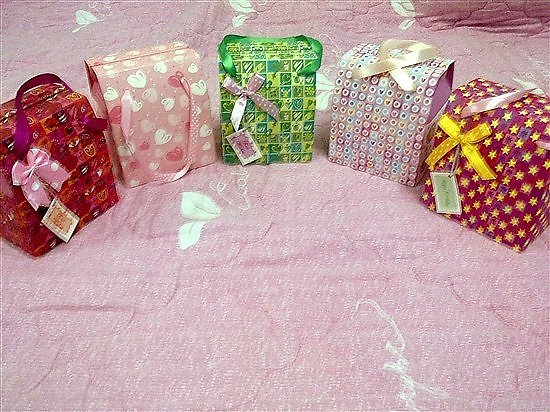The image captures a top-down view of a pink surface, possibly a large blanket or a comforter, featuring a pattern of white leaves and some partial white script starting with "C-O-L." Distributed across the fabric are five distinct gift boxes. 

The first box, red in color, is adorned with a pattern of hearts and features a pink ribbon with white polka dots tied into a bow. It has a deep pink handle and a white name tag accented with pink designs.

Adjacent to it is a light pink box decorated with white, pale pink, and darker pink hearts. This box is finished with a pale pink ribbon handle dotted with white.

Next, a green box presents a grid design with various hearts inside each square and is accentuated by a silver bow with white polka dots. It includes a solid green satin handle and a matching name tag.

The fourth box is lavender, exhibiting a pattern resembling clouds in different shades of blue and yellow, interspersed with multicolored hearts in small white circles. It is complemented by a white satin ribbon handle.

Finally, there is another red box, this one covered in yellow stars and tied with a yellow satin ribbon bow with white polka dots. It has a pale pink satin ribbon handle and a green name tag.

All the packages are neatly arranged on the pink, leaf-decorated fabric, making for a colorful and festive display.